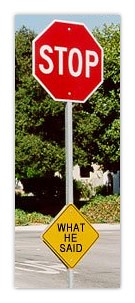The image showcases a distinctive, computer-generated stop sign, distinct from those typically seen on public streets. The red stop sign, affixed to a metal pole, stands prominently in the foreground. Adding to its uniqueness, a yellow, diamond-shaped sign is attached below it, bearing the bold, capitalized text "WHAT HE SAID." This black lettering on a yellow background complements the stop sign while providing a vivid contrast that makes the message conspicuous.

The backdrop features a cluster of large, rounded trees with a lush, bush-like quality, underlined by tall, verdant grass that adds richness to the scene. The setting appears to be a parking lot, suggested by the positioning of the sign. Below the foliage, the bottom segment of a building is partially visible in the background, hinting at an urban context while maintaining focus on the intriguing signage.